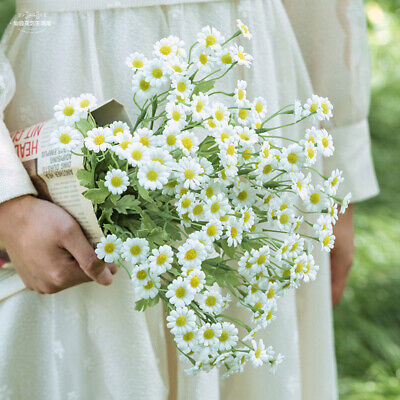In this square image, taken in daytime, we can see the lower part of a person dressed in a white robe or cotton dress. The person is holding a bouquet of small, beautiful flowers with white petals and yellow centers, all bound together with green stems and leaves. The bouquet is wrapped in an old newspaper and is held by the individual's side, near their thigh. The background is blurred, revealing hints of grass and leaves, suggesting a garden or a grassy field. The sunlight illuminates the scene, adding a natural glow. In the top left corner, there is a barely visible logo or watermark, possibly featuring Chinese characters.